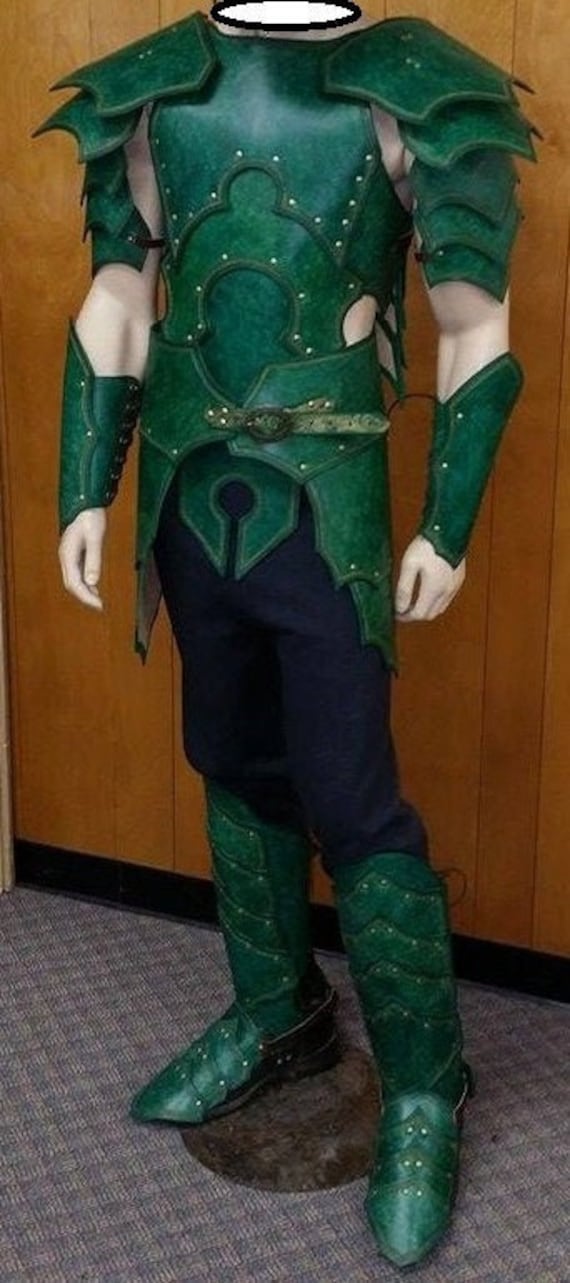The photograph captures a headless plastic mannequin displaying an intricate green superhero outfit within a room characterized by light, neutral-colored wood paneling and a carpet with a bluish-tan checkboard pattern. The mannequin, modeled to resemble Caucasian skin with its pale arms, showcases a detailed ensemble comprising various green hues. The top features layered shoulder pieces and a green breastplate cinched by a central belt. The sleeves consist of arm pieces extending from the wrists to the elbows, marked by openings that provide a textured, layered look. The costume transitions into black pants that are neatly tucked into dark green boots. These knee-high boots exhibit a scaly texture with button-like bolts, evoking an almost reptilian or baby alligator appearance. This meticulously designed outfit, reminiscent of elfin attire suitable for live-action role-playing, exudes an otherworldly charm with its mix of bright and dark green elements.